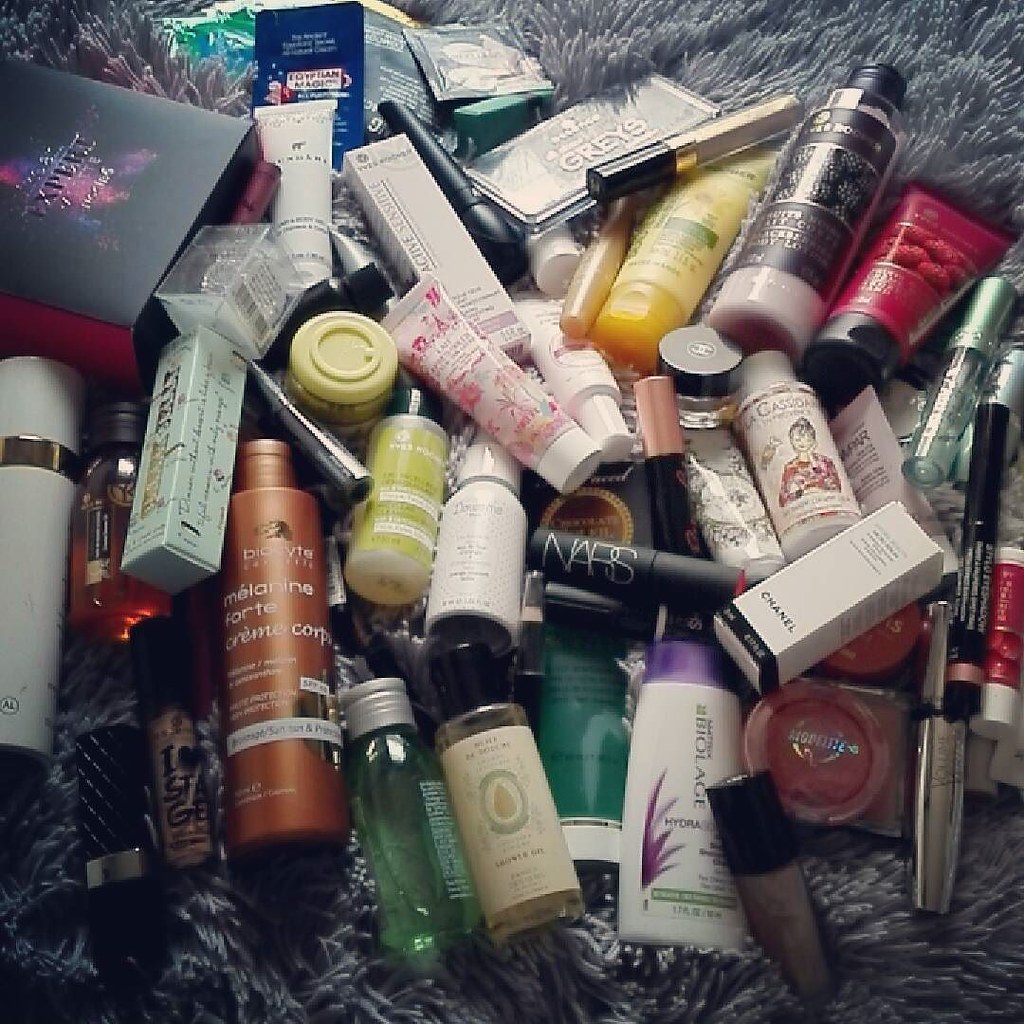The photo depicts a chaotic assortment of beauty items scattered on a plush, gray, furry rug. The image quality is poor, with noticeable blurriness and pixelation, making it difficult to read the text on many of the products. Despite this, a variety of cosmetic and skincare items are discernible amidst the colorful mess.

Prominent among them is a large brown bottle, possibly containing lotion, and a black bottle embellished with blueberry graphics. There's also a distinctive red, triangular container featuring raspberries, likely another lotion. A black cosmetic item, possibly lipstick or eyeliner, is branded with "NARS" in white. Several yellow items, including lotions in yellow bottles and circular containers, stand out in the clutter.

Scattered among these are white boxes and a container featuring a cartoonish depiction of a woman. The collection also includes an eyeshadow palette positioned toward the back right. The overall scene showcases a vibrant mix of reds, yellows, and whites, against the textured rug background.